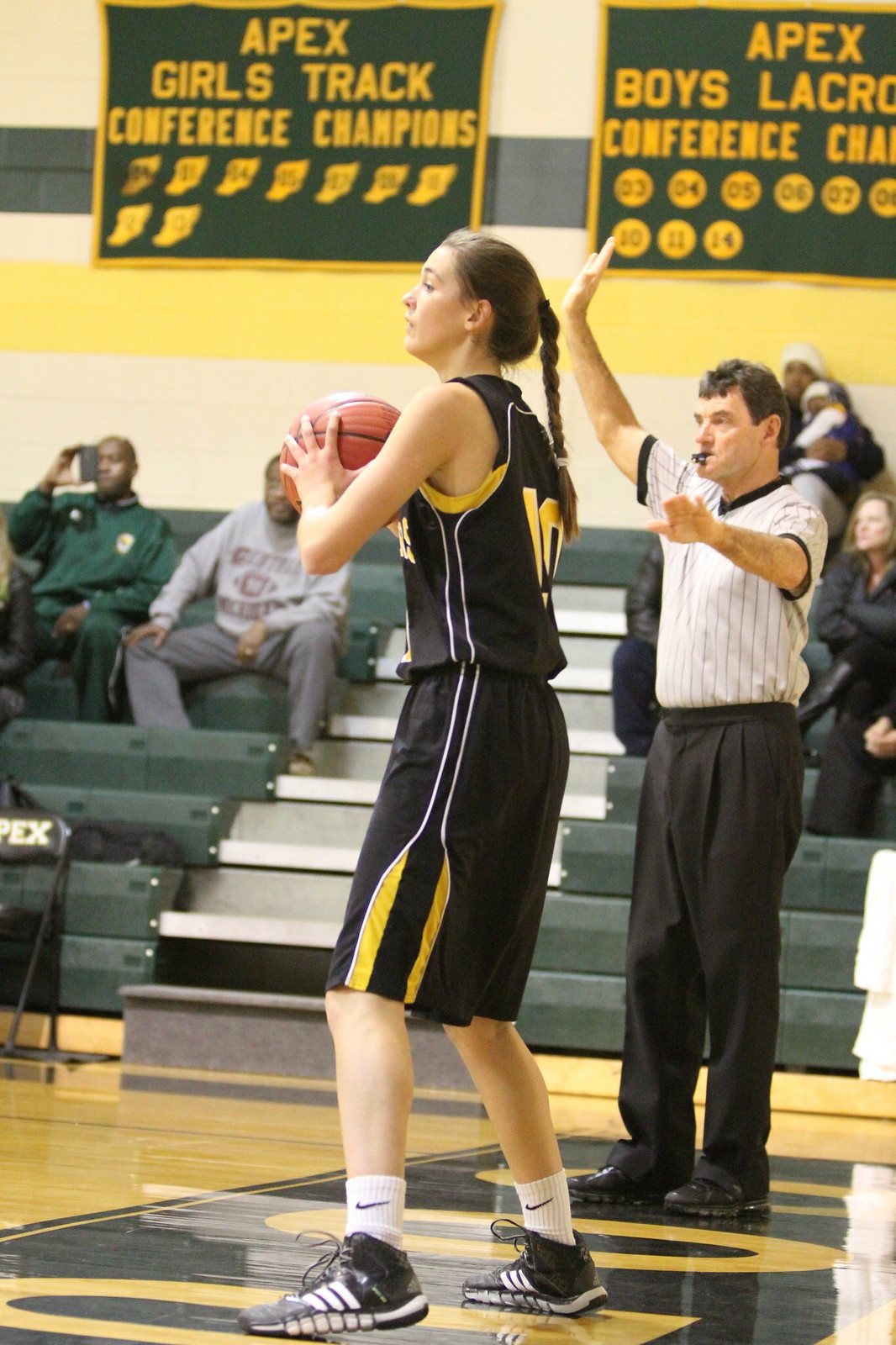In this close-up photo inside a gymnasium, a tall girl with long, braided brown hair is positioned in the foreground, wearing a black basketball jersey and shorts with white and yellow trim. She has on white Nike socks and black sneakers with white stripes. Holding a basketball firmly with both hands against her chest, she stands near the baseline of the court, appearing poised to inbound the ball. Her knees are slightly bent, and her intense focus suggests she might be preparing to make a play.

To her right, a referee is captured mid-action, with his right hand raised and his left arm extended to the side, a whistle in his mouth, wearing a white-striped shirt and black pants. In the background, aluminum bleachers are filled with spectators, including a man possibly taking a picture with his phone and another holding a child. The gym wall is adorned with black and yellow school banners highlighting achievements such as "Apex Girls Track Conference Champions" and "Apex Boys Lacrosse," reinforcing the school pride. The shiny yellow basketball court reflects the dominant black and yellow theme of the surroundings.